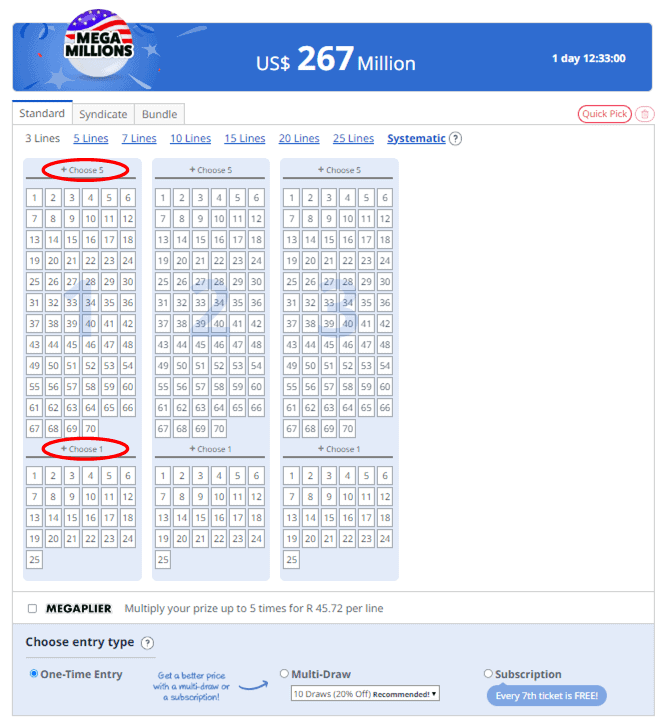This image displays a selection page for the Mega Millions lottery. The top section features a vibrant blue rectangle, with a circle containing an American flag situated in the left corner. Inside the circle, "Mega Millions" is written in black text, accompanied by stars and sparks. Centrally positioned, white text announces the jackpot amount: "U.S. Dollars, $267 million." On the far right, a timer reads "One day, 12:33:00."

Below this, a large white square background hosts three tabs labeled: "Standard," "Syndicate," and "Bundle." To the right, a red-outlined oval with a white background contains the red text "Quick Pick."

Underneath, black text lists various options: "3 lines," "5 lines," "7 lines," "10 lines," "15 lines," "20 lines," "25 lines," and "Systematic?".

Further down, three vertical light blue rectangles display grids of numbers ranging from 1 to 70. The first rectangle has its top section circled in red with the instruction "Choose 5," and its bottom section circled with a red oval stating "Choose 1." The second and third rectangles are similar but lack any circled sections.

Below these number grids, bold black text reads: "Megaplier. Multiply your prize up to 5 times for R4572 per line."

At the bottom, a light blue rectangle spans the width of the image, offering entry type options: "Choose entry type: One-time entry, get a better price on a Fibe [Five?] Draw or a subscription, Multidraw, Subscription."